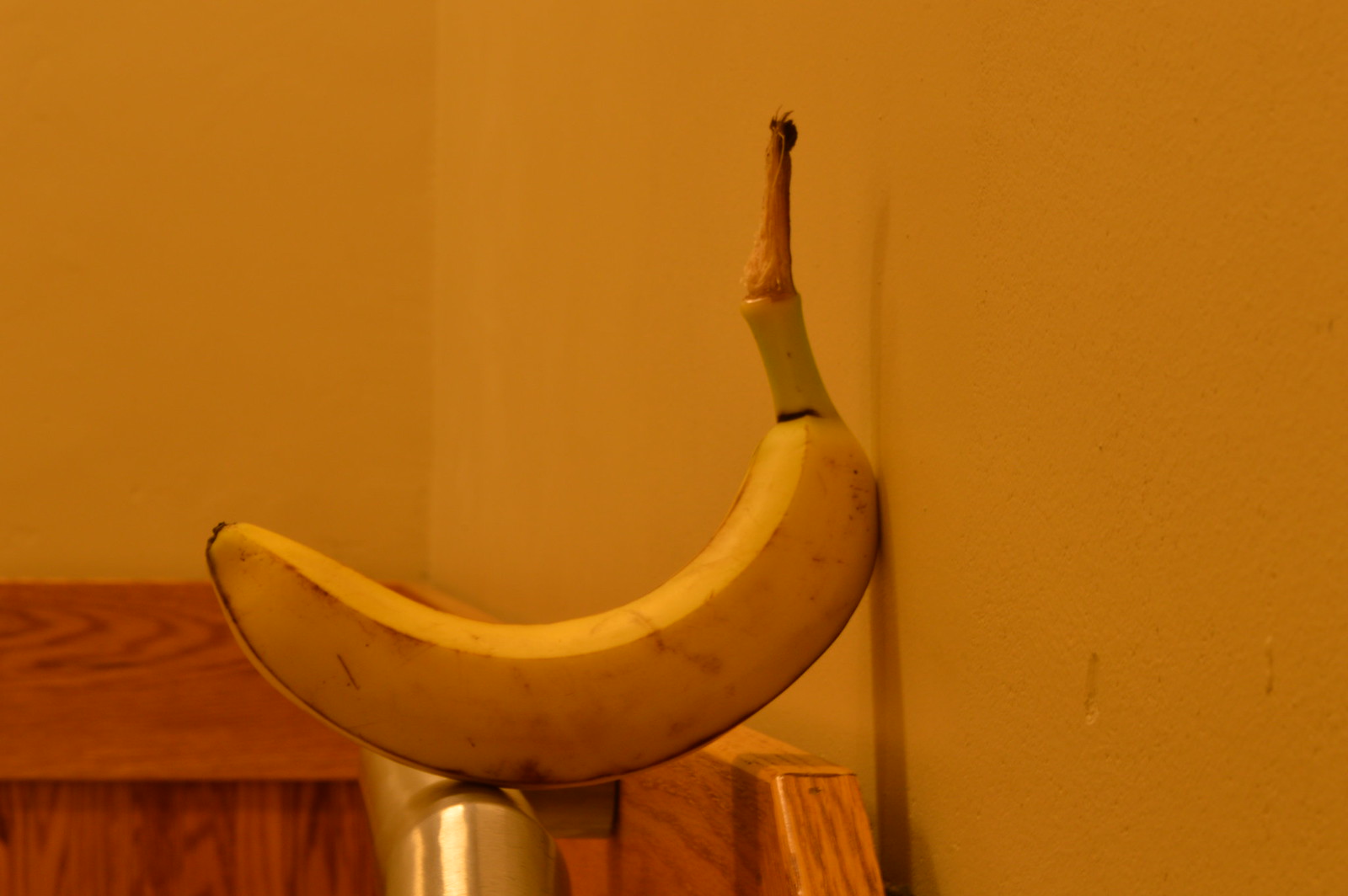In this intriguing photograph, a ripe, unpeeled banana casually rests on a wide brass handrail. The brass handrail is accentuated by a light-colored pine wood trim, which has been treated with a clear varnish to bring out its natural hues. Behind the rail, an orange wall, shaded in a rich, burnt ochre hue, provides a warm backdrop. The banana itself is marked with the telltale black spots and streaks of ripening, indicating its readiness to be eaten. The fruit's stem also shows signs of darkening, adding to the sense of its ripeness. This seemingly mundane yet oddly placed banana invites curiosity, not only about who placed it there but also about the fleeting moment captured in the image before the banana likely resumed its journey with its photographer.